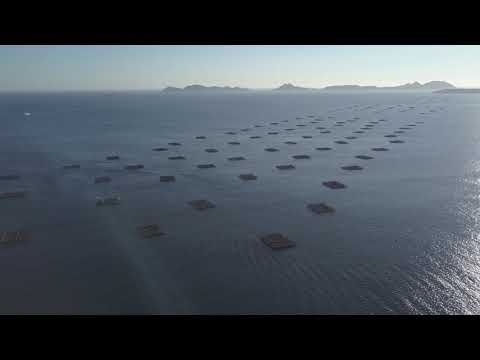This aerial color photograph taken at sunset captures a serene, expansive body of water, possibly an ocean or bay, with a range of blue mountains or islands in the far distance beneath a pale, nearly cloudless sky. The water, which is a dark blue, is dotted with numerous rectangular or square structures floating in its center, arranged in five distinct rows that stretch into the horizon. These structures, around fifty or more, are dark-colored, possibly green, and may be wooden platforms, flotation devices, or part of an aquaculture operation like an oyster farm. The image is rendered in a realistic style, with notable stillness and clarity, and the sun is reflected in the bottom right corner of the water. The photograph's landscape orientation emphasizes the extensive, calm water surface devoid of boats, bordered at the edges by open water contrasting with the clustered central structures, making for a strikingly detailed and tranquil scene.